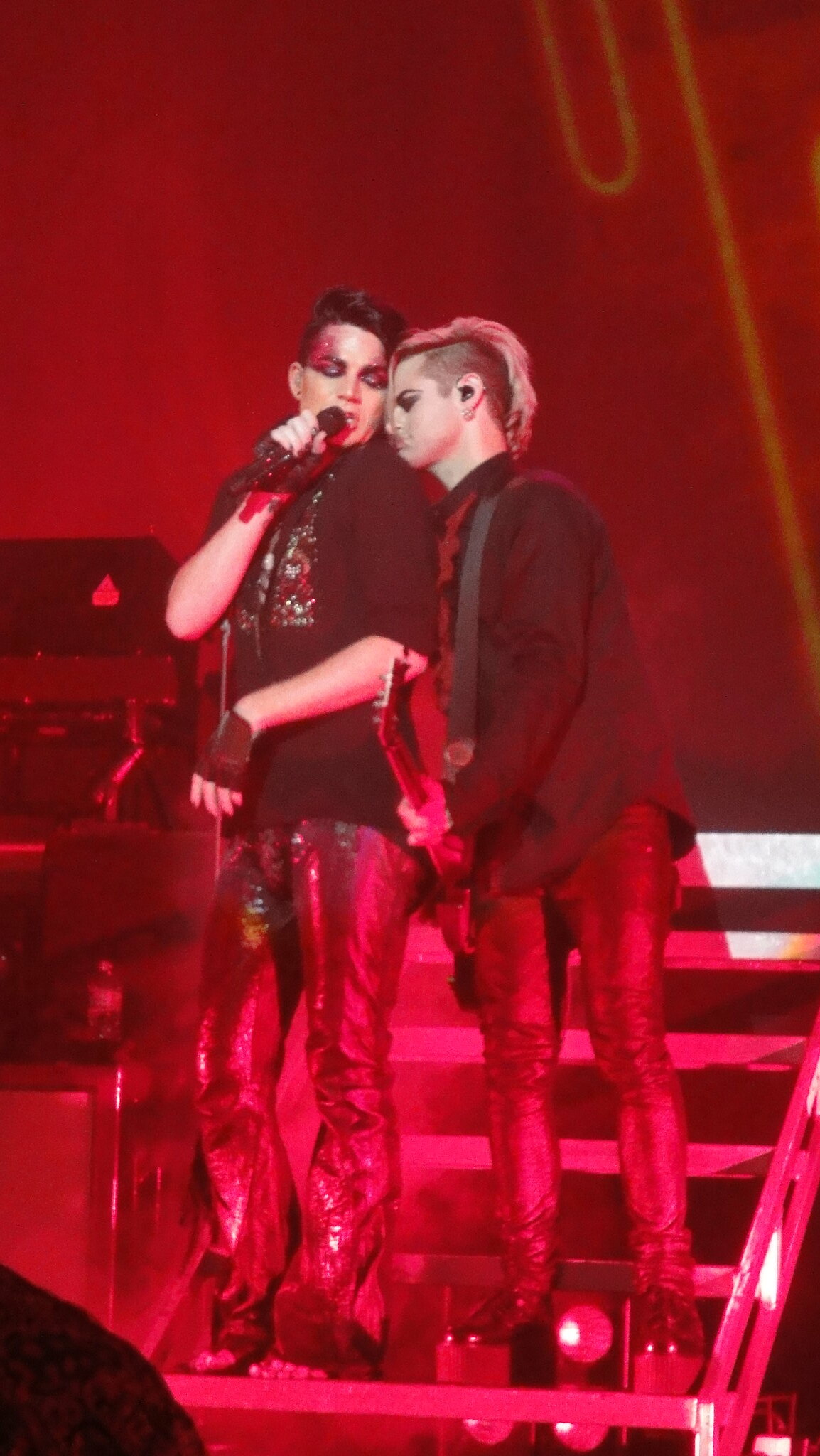The image captures a dynamic performance by two young artists on a six-step stairway, with both occupying the very first step. Dominating the center of the picture, they are enveloped in a dark red hue that casts a dramatic tone over the entire scene. The artist on the left, who appears slightly taller, is singing passionately into a microphone. This vocalist, who has black spiky hair and is dressed in a black t-shirt paired with shiny leather pants, is also wearing gloves. The artist on the right has a distinctive mohawk with shaved sides, possibly blond or gray due to the red lighting. He's deeply immersed in playing his electric guitar, his chin resting on the singer's shoulder and eyes closed. His attire includes a black button-down jacket, white leather pants, and strikingly high black platform shoes with four-inch soles. Both performers exude a punk rock aesthetic, and the stage is illuminated by circular lights beneath the stairs, adding an atmospheric glow to the reddish scene.